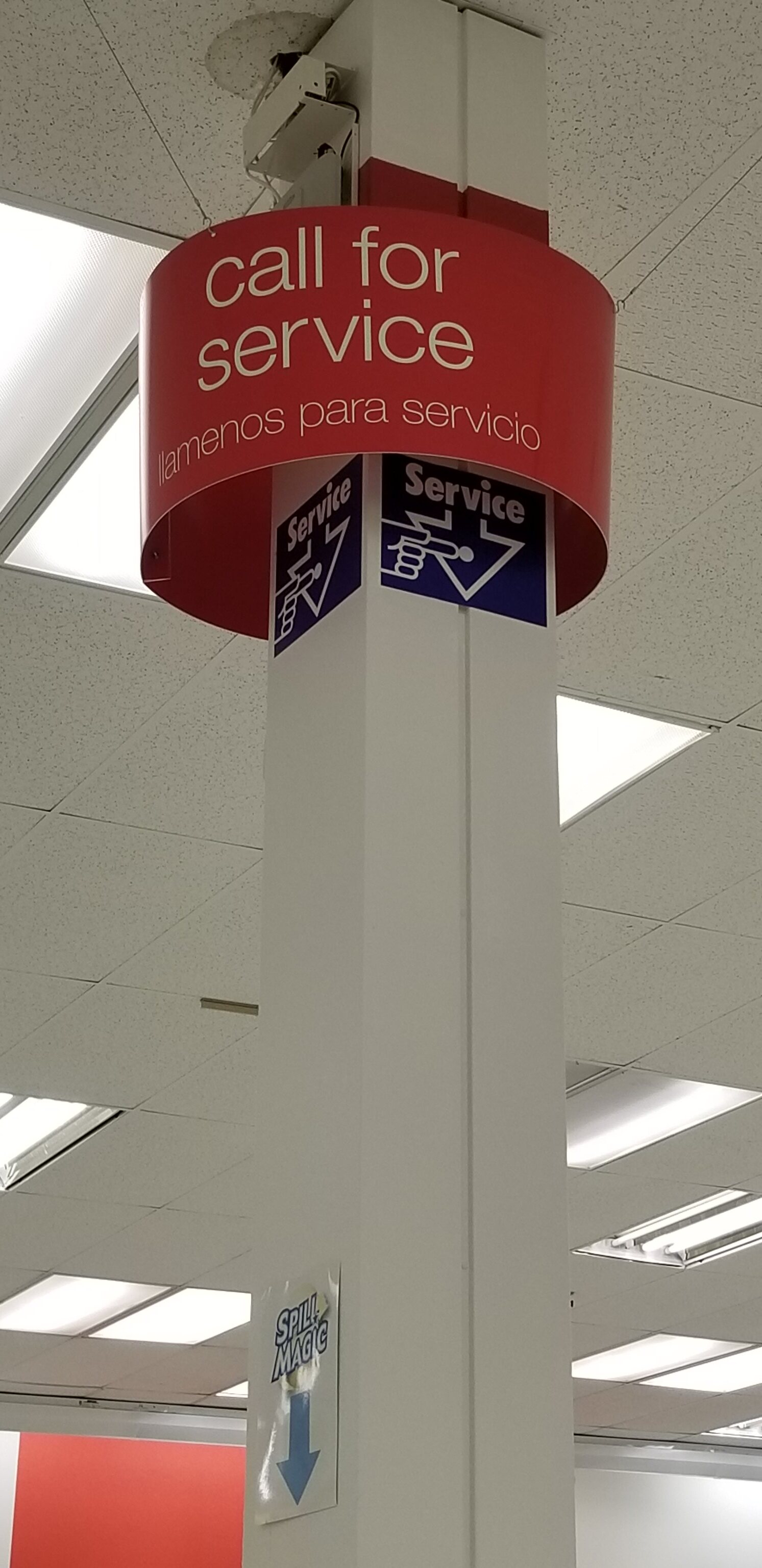Inside a store, the image captures a white rectangular pillar extending from the ceiling to the floor. The ceiling itself is composed of square fiber tiles interspersed with rectangular fluorescent light panels emitting a soft white light. At the top of the pillar, a red circular sign encircles it, bearing the message "Call for Service" in white text, followed by the Spanish translation "Laminos Para Servicio." Affixed to the pillar beneath the red sign are two blue stickers, each with an arrow pointing down and depicting a hand pressing a button. These stickers also bear the word "Service" in white letters. Further down the pillar, there is a laminated white paper sign featuring a blue arrow pointing downward. In the bottom left corner, a red square object, possibly a sign or part of the wall, is visible, partially obscuring the view.